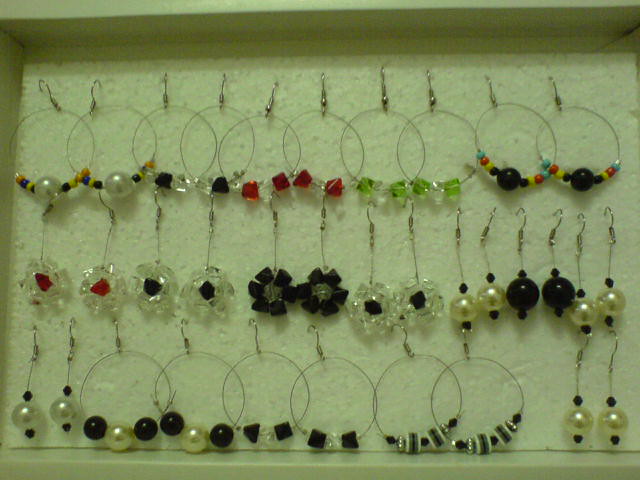This photograph features a detailed display of earrings arranged in a white jewelry box with a cotton insert background. The earrings are meticulously organized into three rows, each showcasing a variety of styles and colors. The top row is predominantly composed of thin metal hoop earrings adorned with various charms, including pearls, gemstones, and different colored beads hanging at the bottom. These beads come in colors like red, black, and clear, with some featuring diamond textures. The middle row shifts towards more intricate designs, with gemstone earrings shaped like flowers, accompanied by pairs of white pearls, black beads that resemble pearls, and more white pearls. The bottom row is a mix, repeating the themes of the top two rows, with thin hoops featuring beads and several sets of dangle earrings, including black, white, clear, and silver beads. Each row spans the full width of the image, creating a cohesive and visually appealing arrangement from left to right.